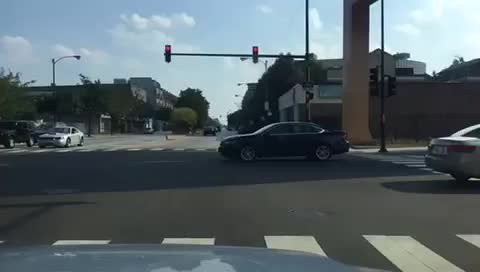This photograph captures a daytime street scene at an urban intersection from the perspective of someone sitting in a light gray sedan, stopped at a red light. The scene showcases a vivid blue sky with scattered white clouds, illuminating the area with sunlight. Traffic lights suspended on a metal bar are prominently visible in the upper third of the image. Directly ahead, the road stretches out, lined with brick buildings on either side. A crosswalk can be seen in front of the car, but there's no pedestrian activity. 

In the intersection, a black sedan rolls from left to right across the street in the foreground, while to the right, the tail end of a silver sedan is visible. On the far side of the intersection, a black SUV and a white Mustang are positioned opposite each other. The dark asphalt road is contrasted by the clear blue sky above, which contributes to the overall brightness of the scene. Light posts and trees are visible in the distance, adding to the urban landscape.